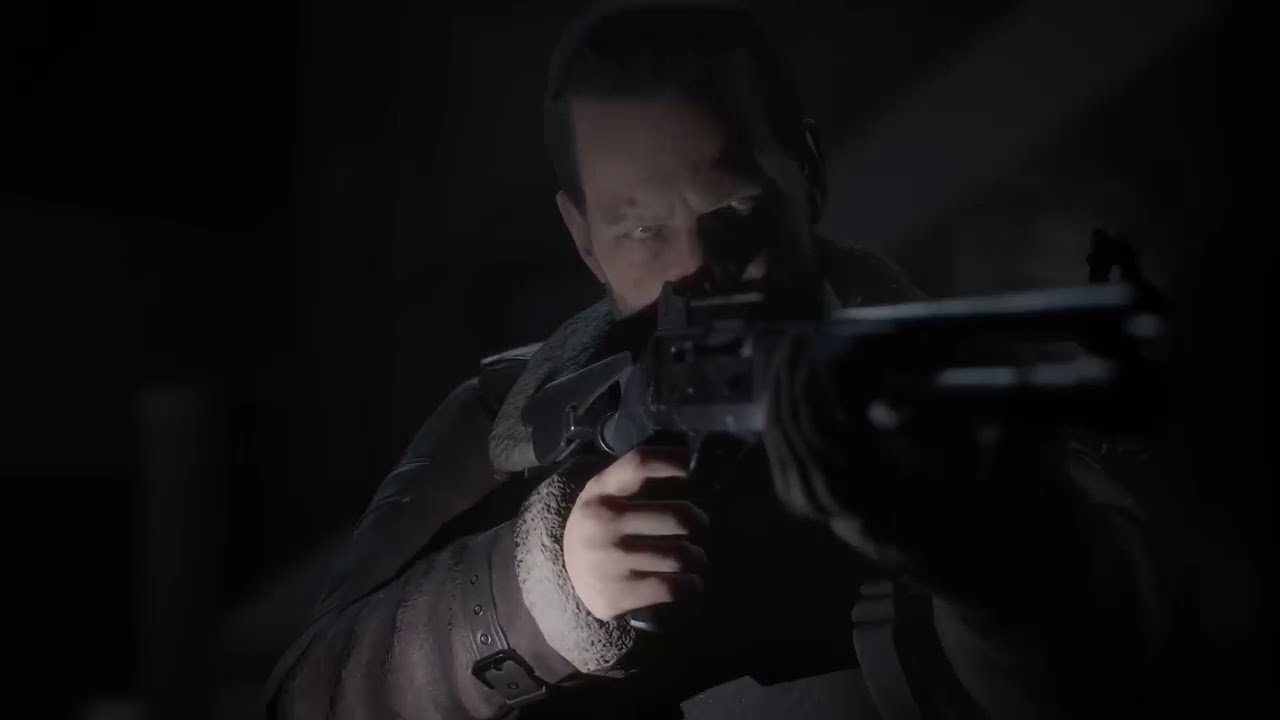The image depicts a close-up of a man holding a large, black, semi-automatic weapon, possibly an assault rifle, against a shadowy and indistinct background. The man wears a heavy winter coat with fur around the collar and cuffs, and a noticeable black leather strap around his wrist. His right hand, visible and gripping the trigger, has fingers teased under the fur cuff of the coat. His left hand, gloved in black, supports the barrel of the gun, though only glimpses of his fingers are visible. The man's face is partially obscured by the weapon, revealing only his intense blue eyes and short hair. The background is completely dark, adding to the menacing and focused expression of the man, who appears poised to take a shot. The overall dark tones of the image, combined with the man’s intent stare and the realistic graphics, give it a video game screenshot feel.